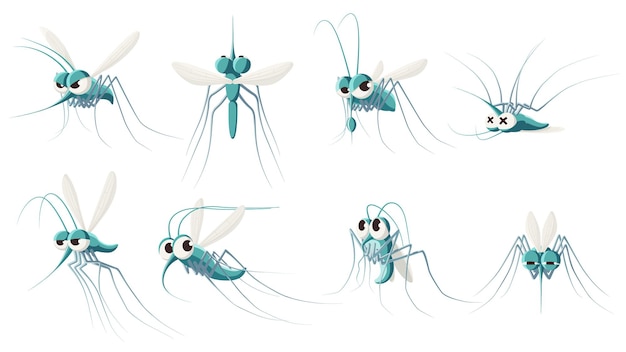This image features a set of eight cartoon-style drawings of turquoise mosquitoes, each depicted in unique positions and emotional states against a plain white background. The mosquitoes are characterized by their oversized eyes, tiny bodies, and very thin legs reminiscent of a daddy long legs, along with protruding tentacles and pointed noses. One mosquito on the top right is illustrated on its back with X's for eyes, indicating it is dead. The top left mosquito has an angry expression, standing upright on all legs. Another nearby mosquito looks upward, possibly having done something mischievous. Among the others, some are flying with tired and scared expressions as if being chased, and one appears cornered, looking fearful. The varied poses and expressions give each mosquito a distinct personality, enhancing the overall whimsical and narrative quality of the artwork.